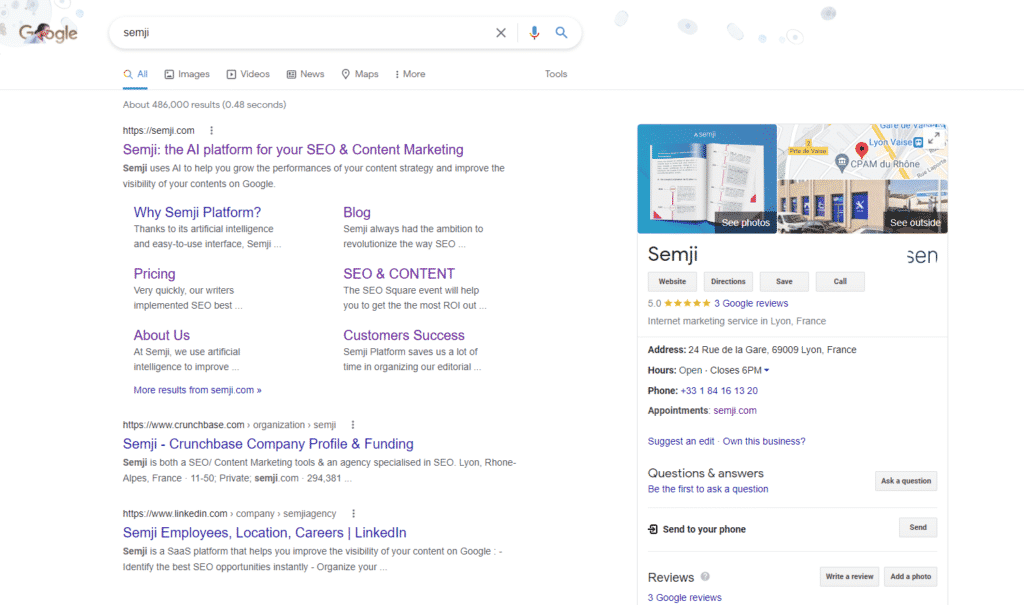**Desktop Screenshot of Google Search Page: A Detailed View of a Search for "SIMG"**

The image captures a desktop screenshot of a Google search page where the user has searched for "SIMG." At the top left, the screen features the iconic Google logo with a special doodle resembling a person's head. The search bar displays the term "SIMG," and the results show approximately 486,000 hits, generated in 0.48 seconds.

Beneath the search bar, options like All, Images, Videos, News, Maps, and More are visible. Additional functionalities such as exiting the search and initiating a voice search are also present.

The first listed result is a website already visited: [SIMG](https://simg.com) - The AI platform for SEO and content marketing. The site description reveals that SIMG leverages artificial intelligence to enhance content strategy performance and improve content visibility on Google.

Next, unvisited links provide more information, although some text is truncated:
- "Why SIMG platform, thanks to artificial intelligence and easy to use interface..." 
- "Blog: SIMG always had the ambition to revolutionize the way SEO..."
- "Pricing: Very quickly, our writers implemented CEO best..."
- "CEO and content: The CEO square event will help you get the most ROI out..."
- "About us: At SIMG, we use artificial intelligence to improve..."
- "Customer success: SIMG platform saves us a lot of time organizing editorial and..."

Additional results include links to:
- [Crunchbase](https://www.crunchbase.com) - The company profile and funding page for SIMG, describing it as an SEO and content marketing tool and agency based in Lyon, France. Notable details: private company, 1150 employees, and the number 294.381.
- [LinkedIn](https://www.linkedin.com) - The company page for SIMG, providing information about employment opportunities, locations, and careers. Description highlights that SIMG is an SAS platform improving content visibility on Google.

On the right, a Google Maps widget displays the location of SIMG. It includes:
- Name: SIMG
- Options: Website, Directions, Save, Call
- Ratings: 5 stars from three reviews
- Business type: Internet marketing service
- Address: 24 Rue de la Gare, 69009 Lyon, France
- Hours: Closes at 6 PM
- Phone number: +33 1 64 16 13 20
- Appointments: Available through their website
- Additional options: Suggest an edit, own this business
- Section for questions and answers, reviews, and photos

Overall, this detailed screenshot provides an in-depth view of search results for the AI-powered SEO platform, SIMG.